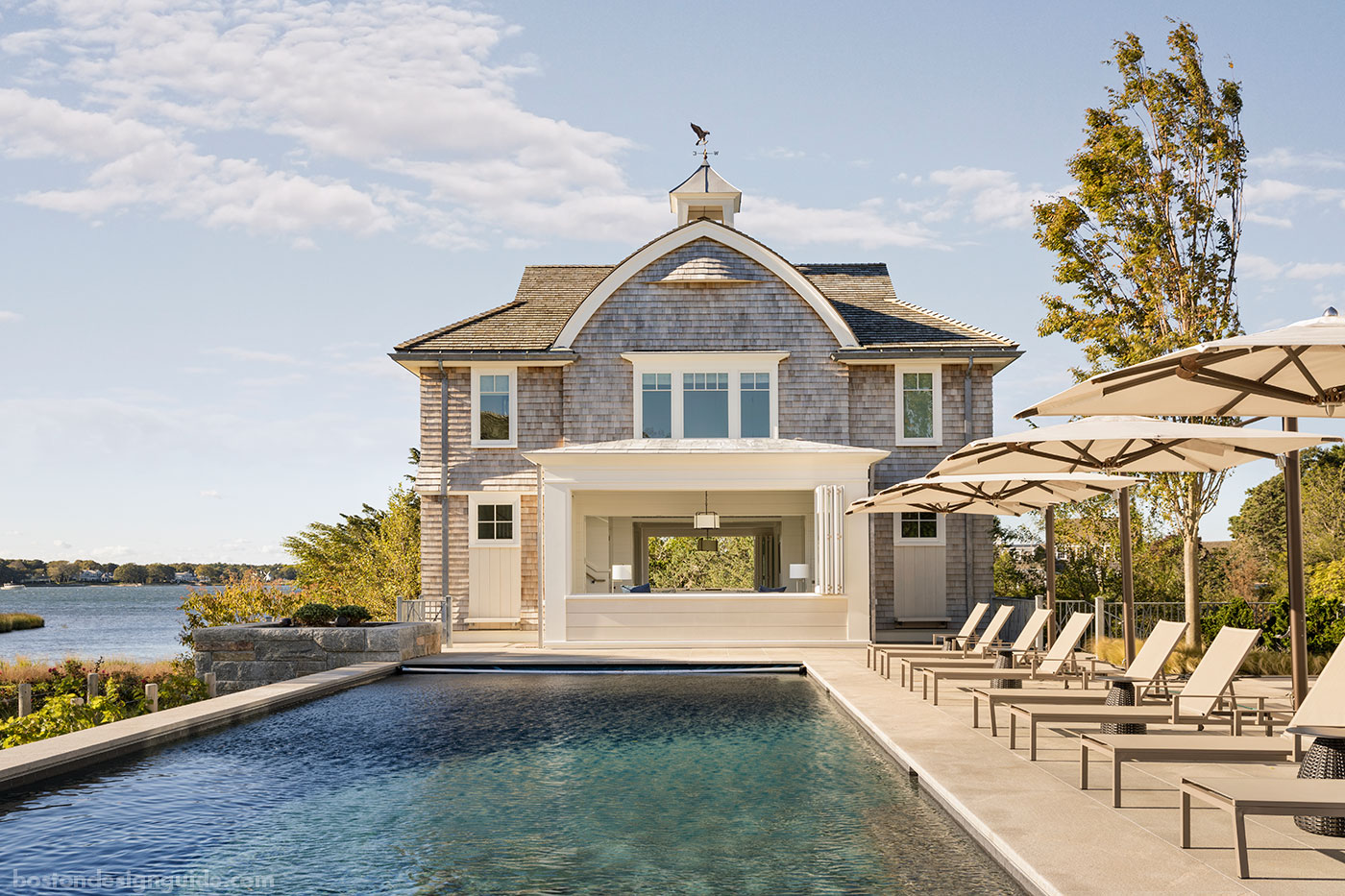In this clear, high-quality photograph, a striking light gray house stands prominently at the center, featuring numerous windows and ample space. The two-story house showcases an open-plan design with a inviting porch and a living room visible from the exterior. The pool, occupying the bottom half of the image, is rectangular, impeccably maintained, and clean. To the right of the pool, a row of light brown sunbeds is lined up, each paired with a matching umbrella providing shade. A tall tree rises behind the sunbeds, adding a touch of greenery and enhancing the summery ambiance.

To the left of the house, the image hints at a scenic lake, creating an intriguing overlap of the pool and natural water body. The backdrop includes a blue sky adorned with a few scattered clouds, further emphasizing the pleasant outdoor setting. Additionally, a watermark reading "bostondesignguide.com" is discretely located at the bottom left corner of the photo. The overall scene exudes a tranquil and luxurious lakeside retreat, perfect for relaxation and enjoying nature.